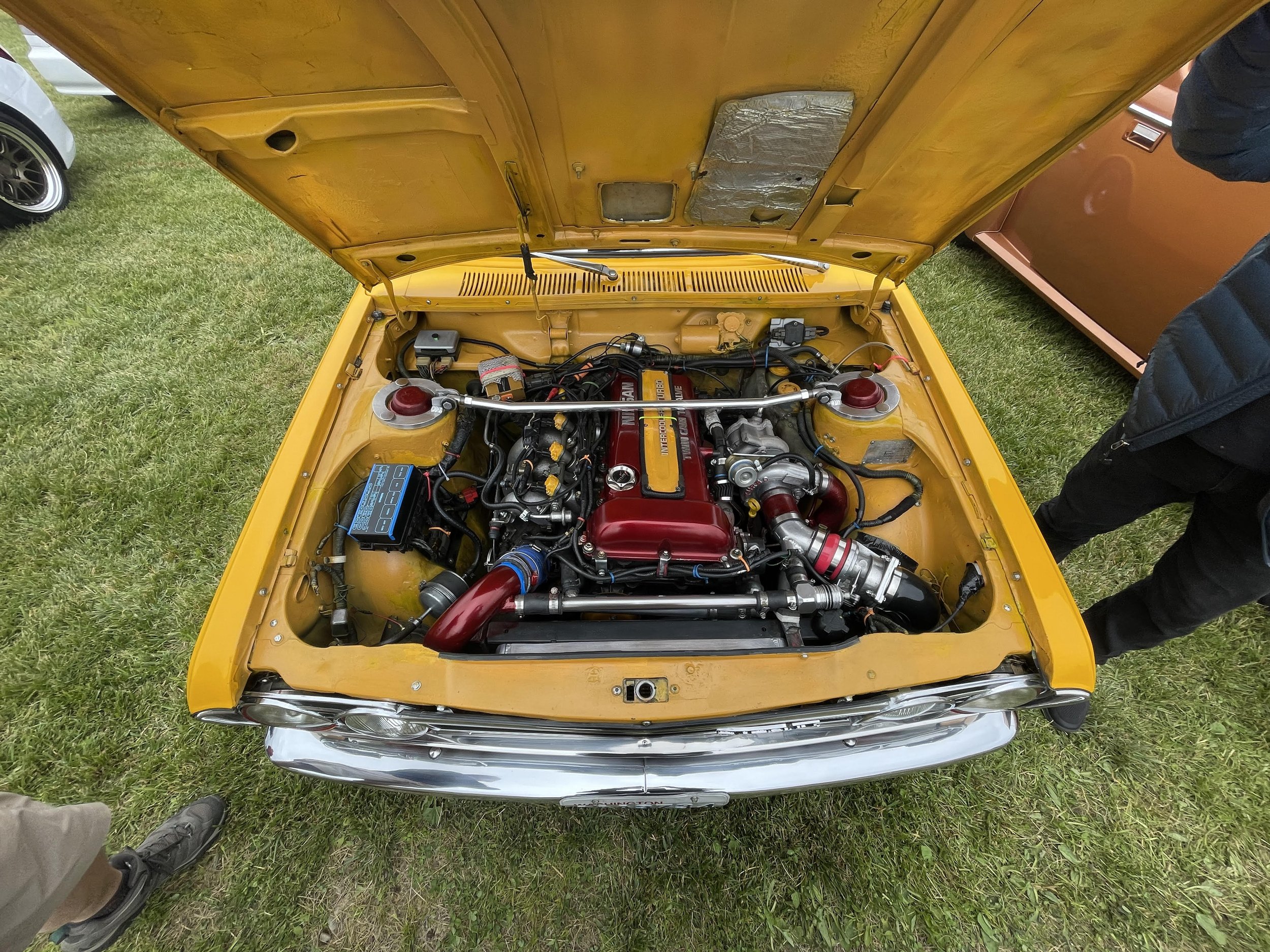This image captures a detailed view of an open hood of a 1970s muscle car, showcasing its powerful and pristine engine. The car features a vibrant yellow-orange paint job, with a strong, clean red engine prominently displaying a Nissan logo and equipped with red valves and pipes. A large silver crossbar spans across the engine bay for structural support. Visible are various engine components, including the battery and spark plugs, set against the backdrop of a shiny chrome grille and bumper, which also displays the vehicle's license plate.

The scene is set at an outdoor car show, as the vehicle is parked on grass with other classic cars nearby; to the right, there's an orange pickup truck and a white car's wheel is visible on the left. The image is taken from the perspective of looking directly down into the engine bay from the hood. Two men are partially visible at the edges of the frame: one on the left in shorts and boots, and another on the right in black pants and a blue sweater.

This striking composition highlights not only the car's impressive engineering but also the nostalgic charm of a classic muscle car enthusiast environment.